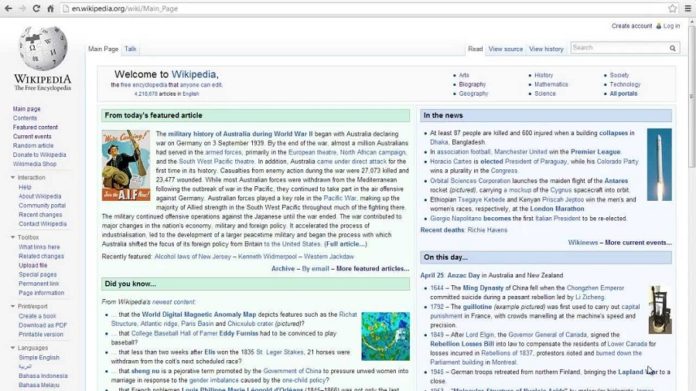This image, sourced from Wikipedia (wikipedia.org), depicts the top portion of the Wikipedia main page. At the very top, it prominently displays the "Welcome to Wikipedia" banner. Just below this section is the "Today's featured article" segment, highlighting information on the Australian Imperial Force (AIF) and the military history of Australia during World War II. The article details how, by the end of the war in 1945, nearly a million Australians had served in the armed forces, mainly in the European, North American, and Southwest Pacific theaters.

Below that, the "Did you know" section features various trivia, accompanied by an image dominated by blue, teal, and green hues. To the right, there is the "In the news" section, shaded in a distinct blue, summarizing the latest news events of the day. Adjacent to this, the "On this day" segment provides historical events and significant dates, offering detailed trivia and information about past occurrences on that specific date.